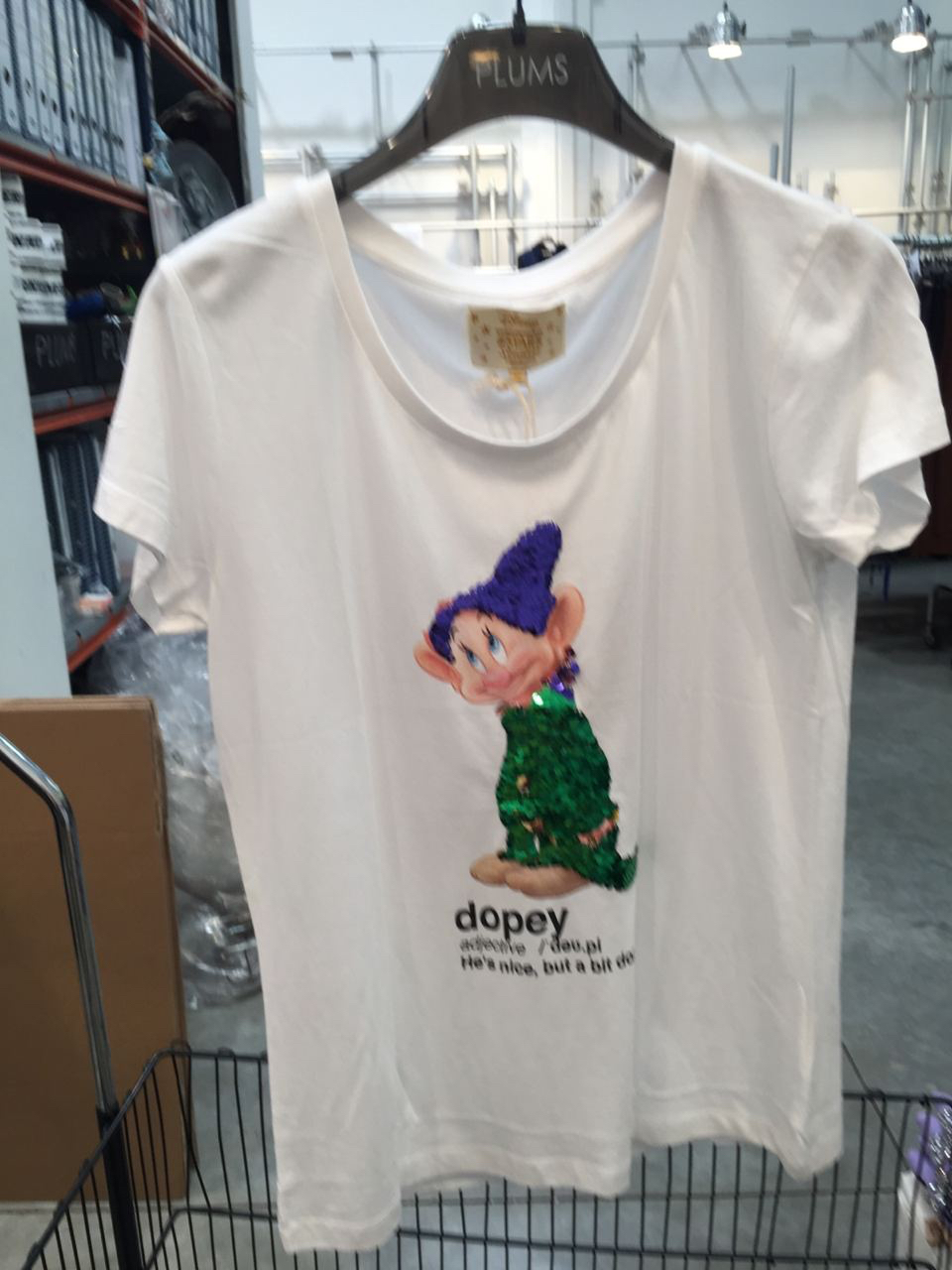This photograph captures a white, slightly wrinkled t-shirt hanging in what seems to be a warehouse or store, evident from the visible shelves, boxes, and black shopping cart below the shirt. The t-shirt is displayed on a black translucent hanger marked with "Plums" across the top, and has a square beige label on its back. The shirt features a detailed graphic of Dopey from Snow White and the Seven Dwarfs in the center of the chest. Dopey is depicted looking to the left, donning a purple sequined hat and a green sequined elf outfit. His ears stick out adorably from the hat, and he has a cheerful facial expression. Below the image, the text reads "Dopey, adjective," followed by its pronunciation. Additionally, it humorously describes him as "He's nice, but a bit dopey." The background shows a concrete floor and more store elements, reinforcing the commercial setting.